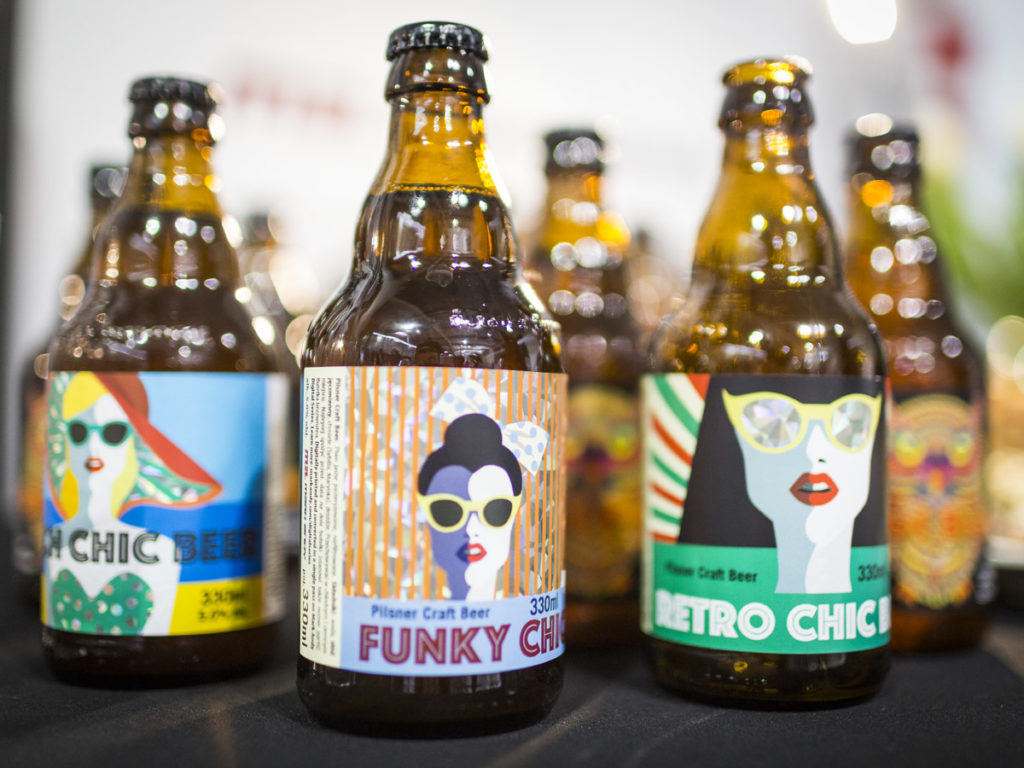The photograph features a close-up of three craft beer bottles prominently displayed in the foreground. Each bottle sports a unique label with artistic illustrations of women, adding a distinct and fashionable aesthetic to the brand. The bottle on the left, labeled "Something Chic Beer," showcases a sketch of a woman in a bathing suit and large floppy hat. The centerpiece bottle bears the name "Funky Chic," with "Pilsner Craft Beer" and "330 milliliters" inscribed above it. Its label is adorned with orange stripes and a stylish woman wearing sunglasses, a dark-haired bun, and a bow tie emerging from the back of her hair. The third bottle, titled "Retro Chic," also carries the "Pilsner Craft Beer" designation. It features a woman with silver and off-white sunglasses, bright red lipstick, and a long white neck. All bottles are capped and filled with a dark yellow or golden liquid. In the background, additional bottles are partially visible, reflecting light that suggests a bright light source to the rear right of the image. This vibrant and chic craft beer presentation emphasizes the brand's indie appeal, potentially resonating well with consumers drawn to its colorful and trendy design.